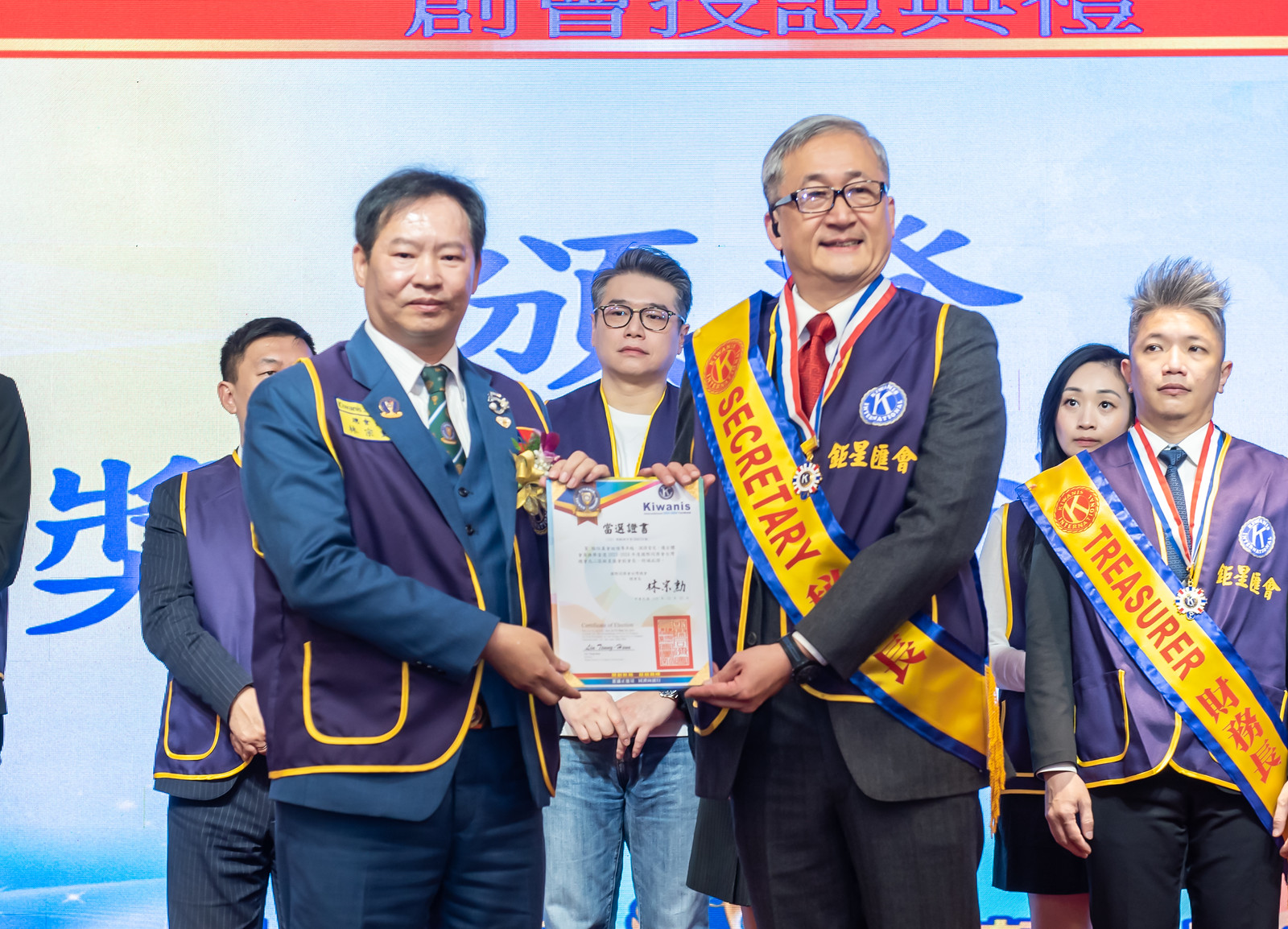The image depicts a group of six individuals, all of whom appear to be members of the Kiwanis club in an Asian country, possibly China, as indicated by the blue Chinese text in the background. They are standing on a red stage with a visually striking red, white, and blue backdrop. Two of the men at the front are holding a distinguishing certificate adorned with decorative elements in blue, red, and yellow. Both men wear blue suits with vests that feature Asian writing and a circular emblem with a 'K'. The man on the left, identified as the secretary, has a yellow sash with a black border and a medal. The man on the right, labeled as the treasurer, has a similar sash. Behind them stands a younger man with black glasses and slicked-back hair, wearing casual jeans paired with a Kiwanis vest. To the left is a man in a blue pinstriped suit and to the right, a man sporting a gray suit with a red tie. A woman in the back, wearing what appears to be shorts or a skirt and a Kiwanis vest, completes the group. This elaborate setup and attire highlight the formal and celebratory nature of the event.